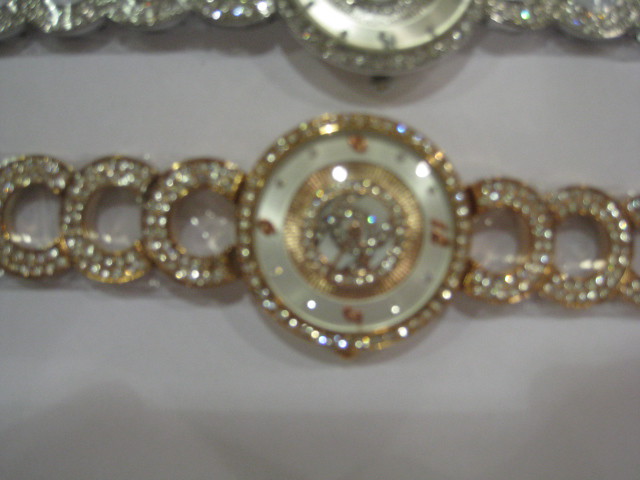An elegantly styled, close-up photograph captures two luxurious women's watches. The primary focus of the image is a gold watch positioned horizontally at the center. It boasts a lavish array of diamonds encircling the entire gold-trimmed face, and the ivory watch face features gold numerals at the 12, 3, 6, and 9 o'clock positions. The design of the band is particularly eye-catching, with interlinked loops that resemble a series of seashells or horseshoes. Above the gold watch, a silver version of the same model is partially visible, also lying horizontally. This silver watch mirrors the gold one's elaborate design, with diamonds encrusted around the face and along the band's edges. Both watches rest on a pristine white background, emphasizing their luxurious appeal and intricate details.